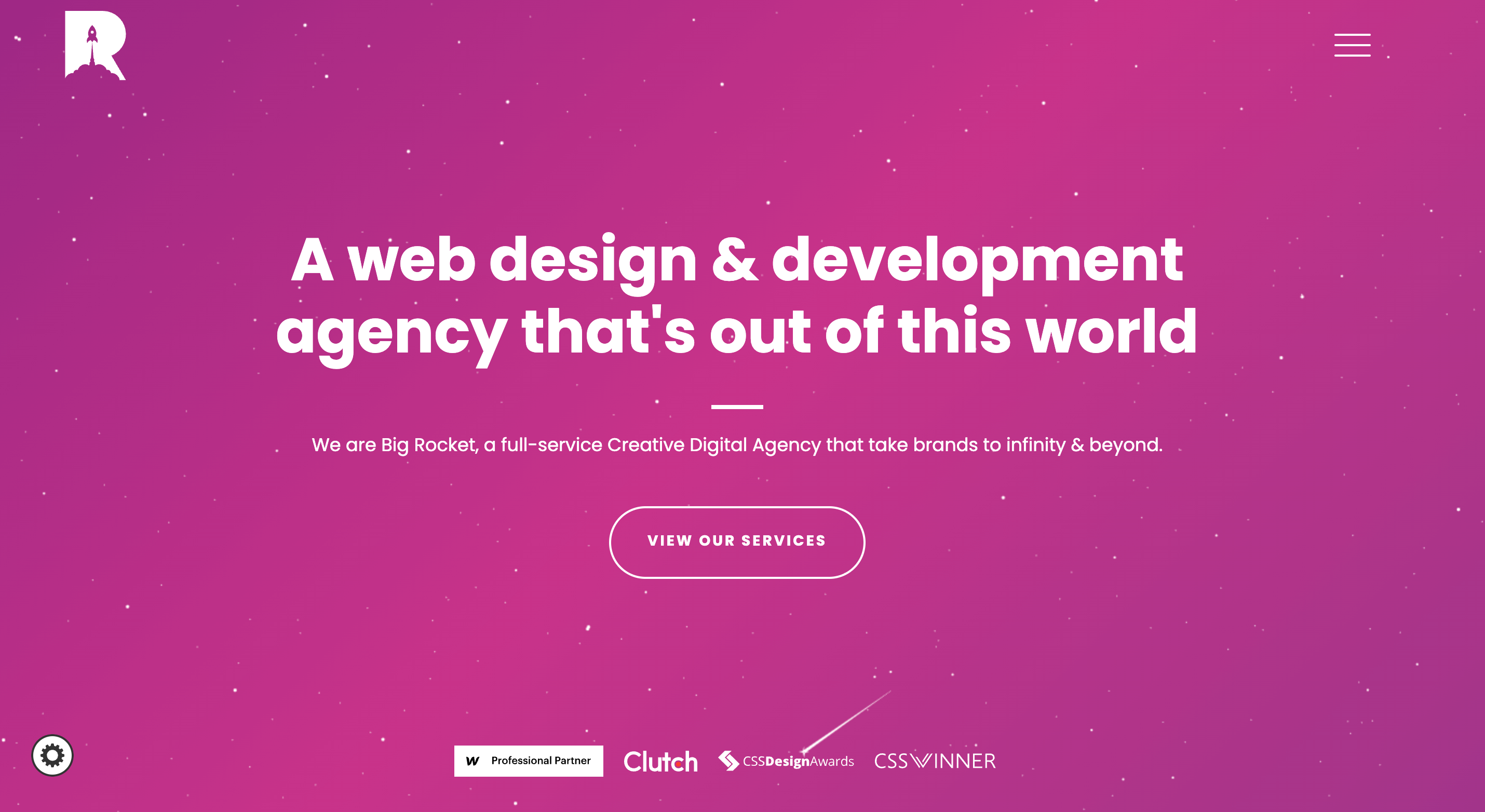**Detailed Caption for the Advertisement Image:**

The advertisement features a company named "Big Rocket" showcased on a vibrant purple background. Dominating the center of the ad is a bold, white text headline: “A web design and development agency that's out of this world.” Just beneath this headline, a thin white line separates it from a smaller text block which reads: “We are Big Rocket, a full-service creative digital agency that takes brands to infinity and beyond.”

Further down, there is a prominent, clickable button in all capital letters stating, “VIEW OUR SERVICES.” At the very bottom of the page, four category icons are displayed in a horizontal line. The first icon represents a "Professional Partner," followed by "Clutch," then "CSS Design Awards," and lastly, "CSS Winner."

In the upper-right corner of the image, a sandwich menu icon is visible, consisting of three white lines stacked vertically, suggesting a drop-down menu upon interaction. Adjacent to this is the Big Rocket logo, creatively designed as the letter 'R' featuring a retro-styled spaceship. The rocket's exhaust forms the legs of the 'R,' while the rocket itself shapes the central circle within the 'R.'